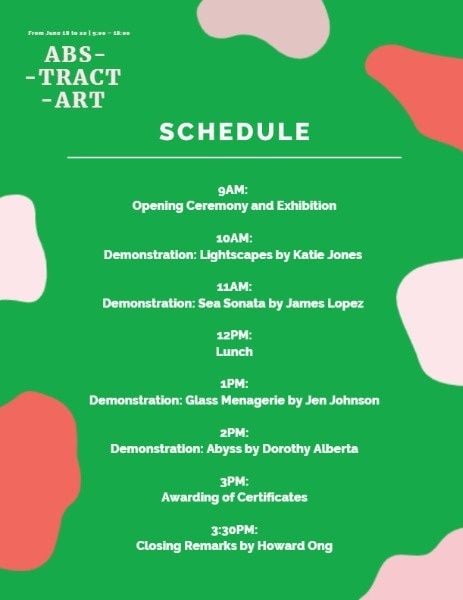The image depicts a green flyer or poster with an abstract design featuring spots or blotches in red, white, and pinkish colors, resembling the patterns found on cows or Dalmatians. These spots are scattered irregularly across the background. In the upper left-hand corner, the text reads "ABS Trapped Art," centered. Below that, the word "Schedule" is boldly underlined. The flyer then lists the event's itinerary: 

- **9 a.m.** Opening Ceremony and Exhibition
- **10 a.m.** Demonstration "Lightscapes" by Katie Jones
- **11 a.m.** Demonstration "Sea Sonata" by James Lopez
- **12 p.m.** Lunch
- **1 p.m.** Demonstration "Glass Menagerie" by Jen Johnson
- **2 p.m.** Demonstration "Abyss" by Dorothy Alberta
- **3 p.m.** Awarding of Certificates
- **3:30 p.m.** Closing remarks by Howard Ong

The flyer effectively presents the schedule for a detailed and engaging day of art demonstrations and events.